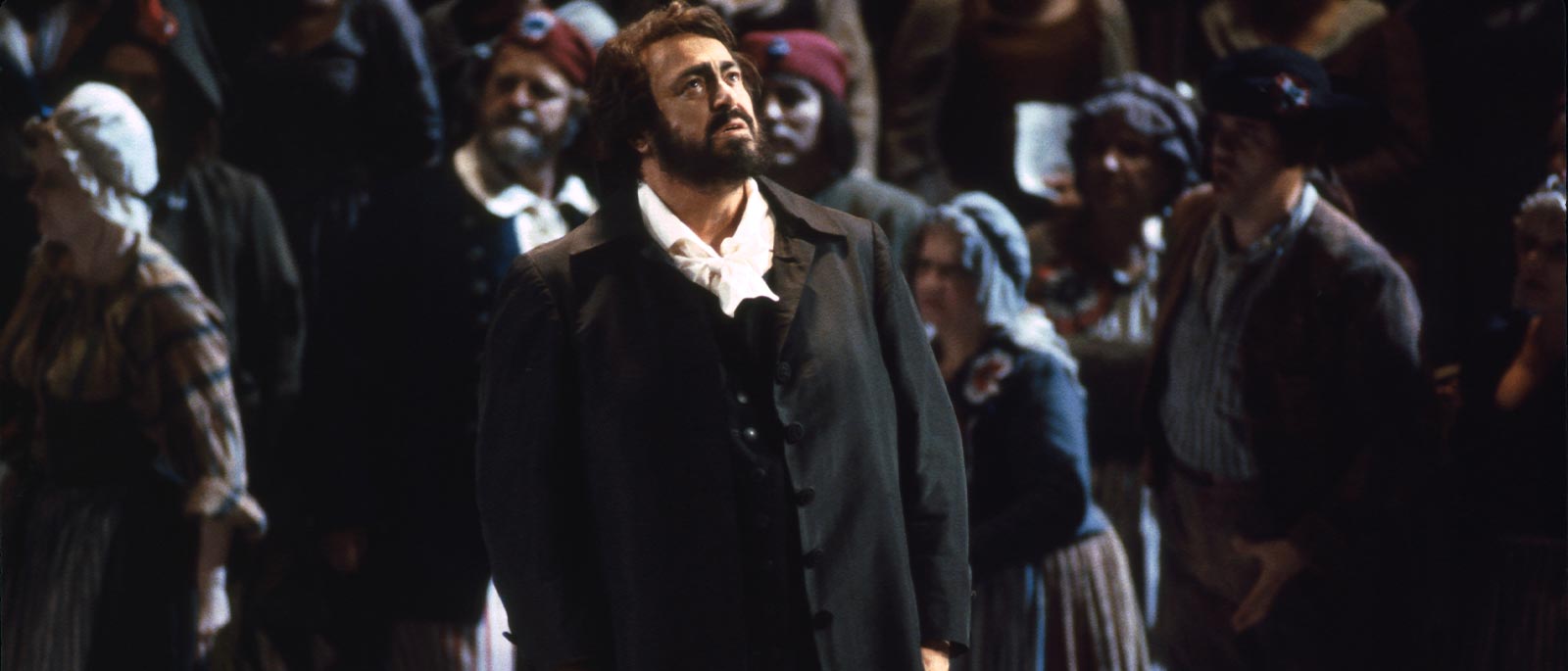In this evocative photograph, reminiscent of a movie scene or opera production, the renowned opera singer Luciano Pavarotti stands at the center, capturing the viewer's attention. Pavarotti, dressed in a black coat layered over a black vest and white undershirt, with his distinctive long hair and thick beard, gazes upwards towards the right with a mixed expression of surprise and sadness. His arms are positioned at his sides. The background features a blurred crowd, consisting of both men and women clad in early 20th-century or late 19th-century attire, seemingly moving towards the left. The photo incorporates a color palette of blacks, whites, blues, light blues, and grays, creating a timeless and somewhat mysterious atmosphere. The image's setting is ambiguous, possibly indoors or outdoors, and it remains unclear whether it was taken during day or night. The collective attention of the figures in the background, contrasting with Pavarotti's upward gaze, hints at an unseen yet significant element above or behind him, deepening the intrigue of the scene.